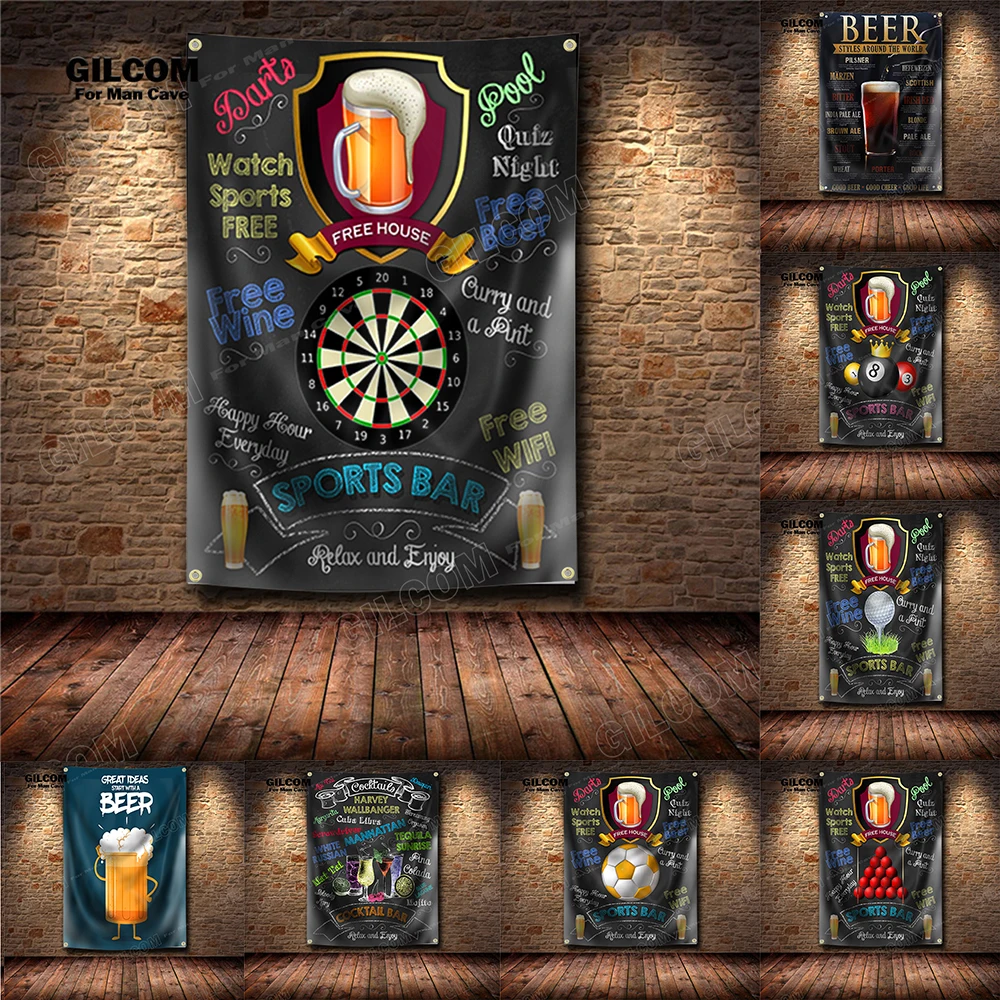The image features a well-decorated stage promoting Gilcom for Man Cave, adorned with various banners and posters centered around a sports bar theme. Dominating the upper left is a large banner displaying an overflowing beer mug and a dart board, surrounded by text such as “Darts,” “Pool,” “Watch Sports Free,” “Free Wine,” “Sports Bar,” “Relax and Enjoy,” “Free Wi-Fi,” and “Happy Hour Every Day.” Flanking this main banner on the right are three smaller ones: the top depicts a glass of dark beer and reads “Beer Styles Around the World,” the middle showcases pool balls and a beer mug with texts like “Sports Bar” and “Free Wi-Fi,” and the bottom features a golf ball on a tee and a beer mug with the label “Sports Bar.”

The lower part of the image displays four additional smaller banners. From left to right: the first is a cartoon beer mug with the phrase “Great Ideas Start With a Beer,” the next is crowded with names of various cocktails including “Harvey Wallbanger,” “Tequila Sunrise,” “White Russian,” and “Manhattan,” alongside the words “Cocktail Bar” and “Relax and Enjoy.” The third banner shows a soccer ball and a beer mug above the words “Sports Bar,” and the last one on the far right portrays a pool rack with a beer mug on top and the labeling “Sports Bar.” The entire scene is set against a dark rustic brick wall and aged wooden planks, adding to the bar's cozy, inviting atmosphere.